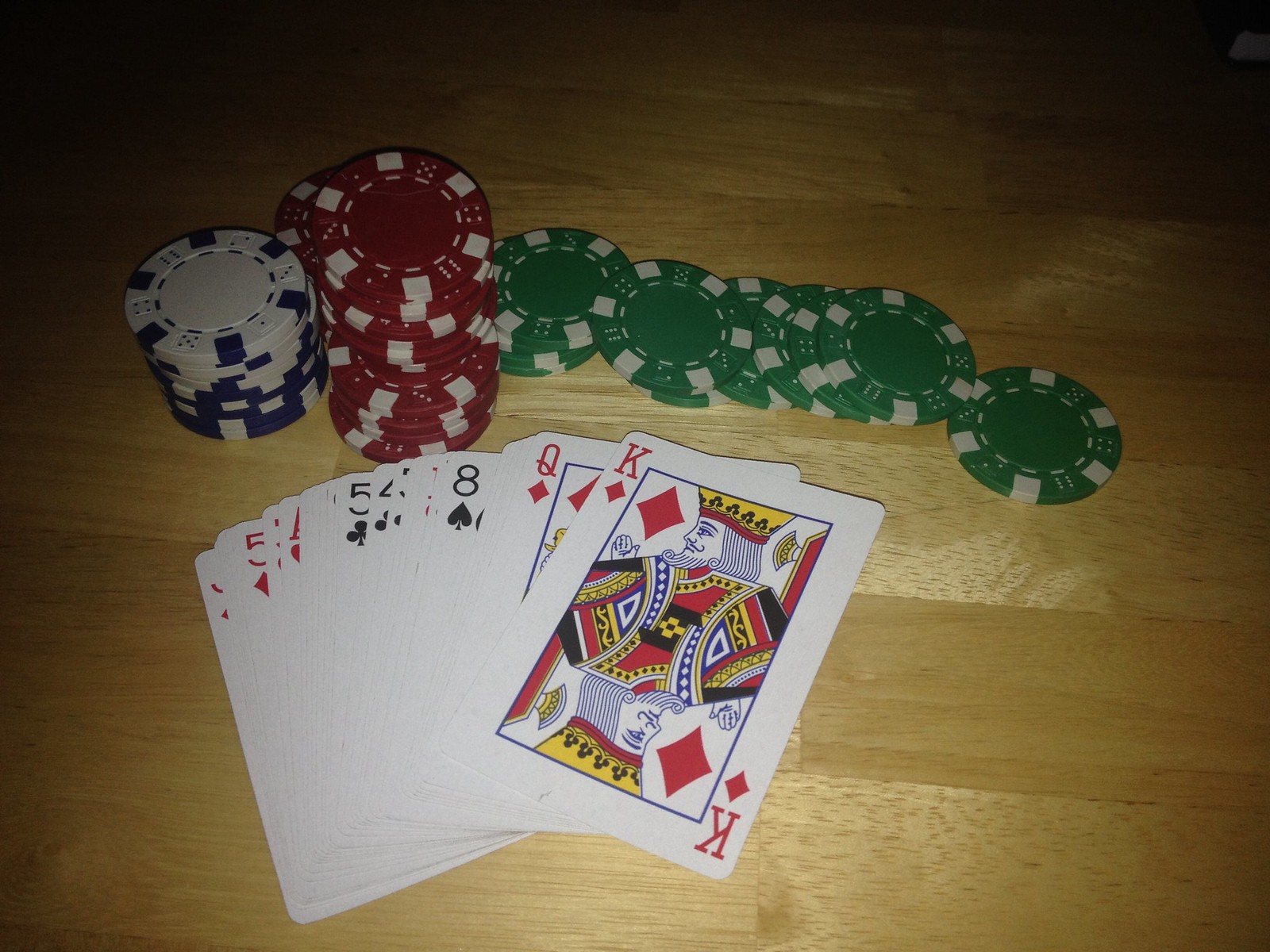An indoor color close-up photograph captures a light tan wooden table from above, displaying a variety of poker accessories in vivid detail. In the upper half of the image, a neatly arranged stack of poker chips spans horizontally. Starting from the left, there is a column of six white poker chips adorned with blue squares around their edges. Adjacent to this is a disorganized stack of red chips, similarly decorated with white squares. Extending from the middle to the right, seven or eight green chips are spread out horizontally, each featuring white squares around their circumference.

In the lower half of the image, several playing cards lie face up, fanning out from the lower left toward the center. Among the visible cards, there is a red five of diamonds, a five of clubs, a four of clubs, an eight of spades, followed by a queen of diamonds. Dominating the arrangement is a king of diamonds positioned slightly diagonally, with the top corner pointing to the upper right. The cards and chips create a vibrant display against the tan wooden background. The upper portion of the image is notably darker compared to the bottom, adding depth and contrast to the scene. No words, text, or additional print are visible in this photograph.